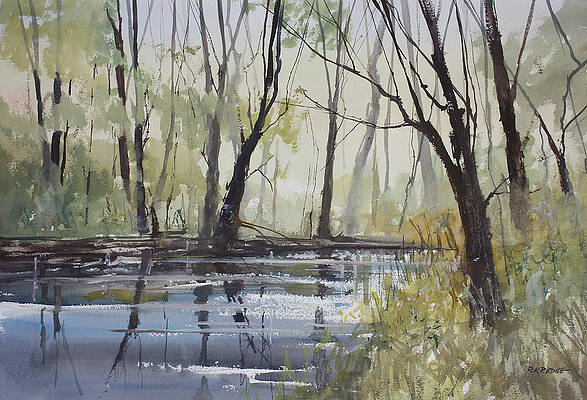The image is a watercolor painting of a serene forest scene, presented in landscape layout. The painting captures a marshland or wetland forest with meticulous detail. The lower left-hand quadrant depicts a tranquil blue pond, its still waters mirroring the surrounding landscape. Reflected in the water are the brown and dark brown trunks of the sparse trees, as well as hints of green foliage. The lower right-hand quadrant reveals a grassy bank adorned with greens, yellows, and browns, along with a prominent tree trunk devoid of leaves but with branches extending outward. The entire upper half features a dense forest with a variety of trees and branches, punctuated by vibrant greenery and peeks of blue and yellow sky filtering through the leaves. A faint, foggy atmosphere permeates the background, adding an element of mystery to the distant woodlands. Despite the minimal foliage on the tall, thin trees, some greenery persists, particularly in the reflections seen in the pond's calm waters.